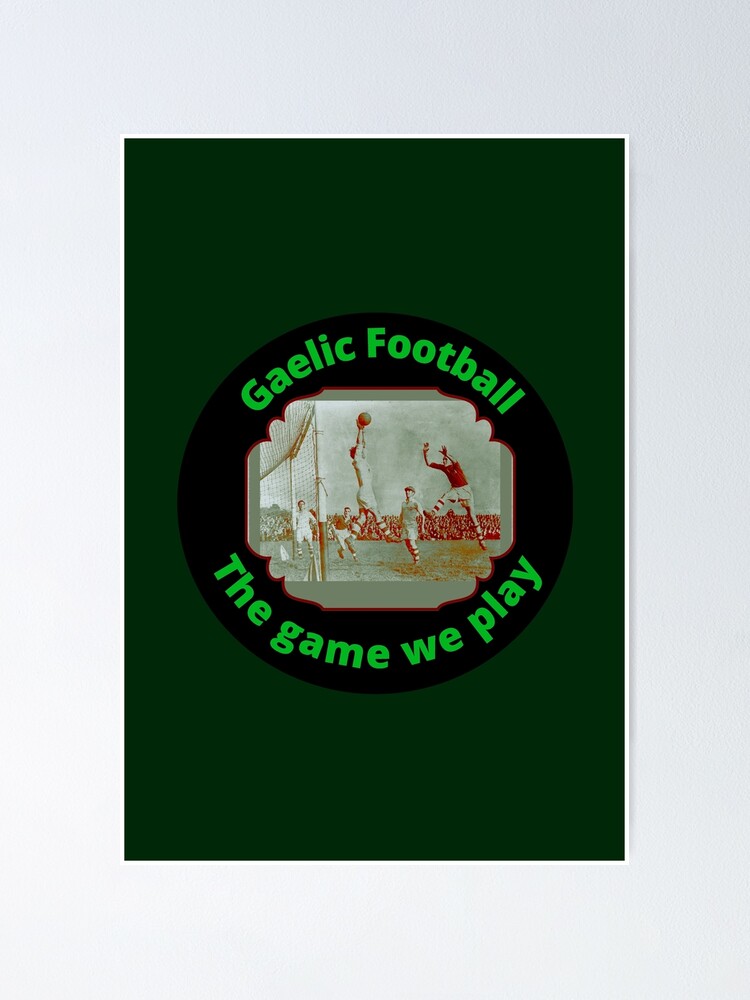The image is a dark green banner or poster featuring a vertical brown rectangle at the center. Within this rectangle, there is a perfect black circle with a grayscale photo of what appears to be an old soccer match. The photo shows several players on the field, with a prominent player in the center jumping with both feet off the ground and hands above his head, seemingly hitting or pushing a ball. There are other players around him, some in light-colored tops and others in darker tops, with one player in red facing him, also airborne with hands raised. Behind the players, a net and distant spectators are visible. At the top of the black circle, in light green text, it reads "Gaelic football," and at the bottom, it says "the game we play." The background of the entire image has a lighter green hue, contrasting with the darker central elements.